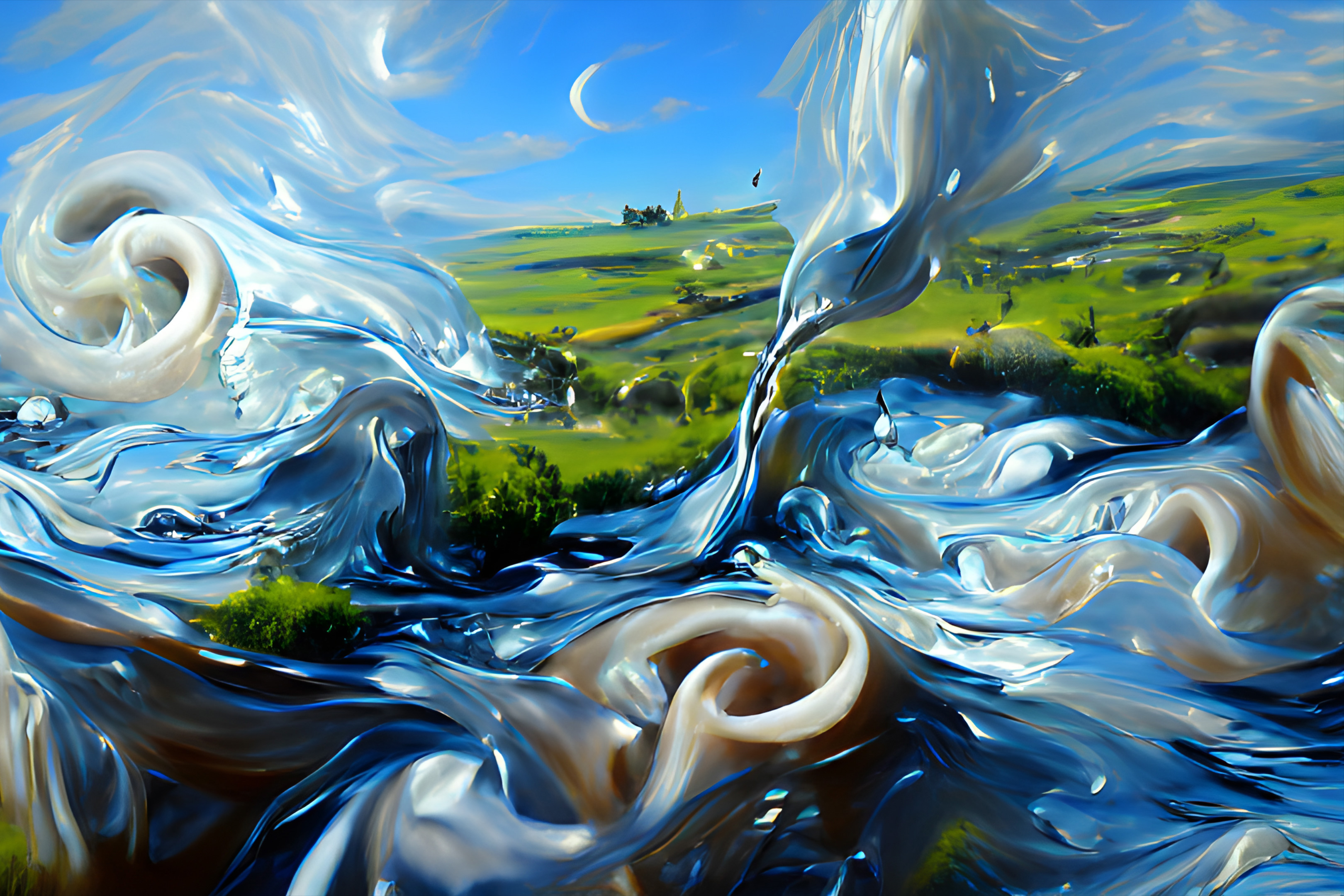The painting showcases a surrealist landscape divided into three distinct sections that seamlessly merge together. Dominating the bottom half of the image is a tumultuous body of water, characterized by its silver metallic sheen and energetic white swirls that seem to defy gravity. These dynamic, swirling waves of water rise from the ground, partially engulfing the green landscape in the midsection. The green landscape itself is dotted with indistinct trees and small, rectangular buildings that are difficult to discern due to their distance. At the top of the painting, a tranquil blue sky is punctuated by a slender crescent moon nestled in the center. The water appears to twist and ascend towards the sky, creating a mesmerizing blend of fluid motion and static elements. The entire composition converges to form a dreamlike scene where the boundaries between water, land, and sky blur, emphasizing the surrealist theme of the artwork.